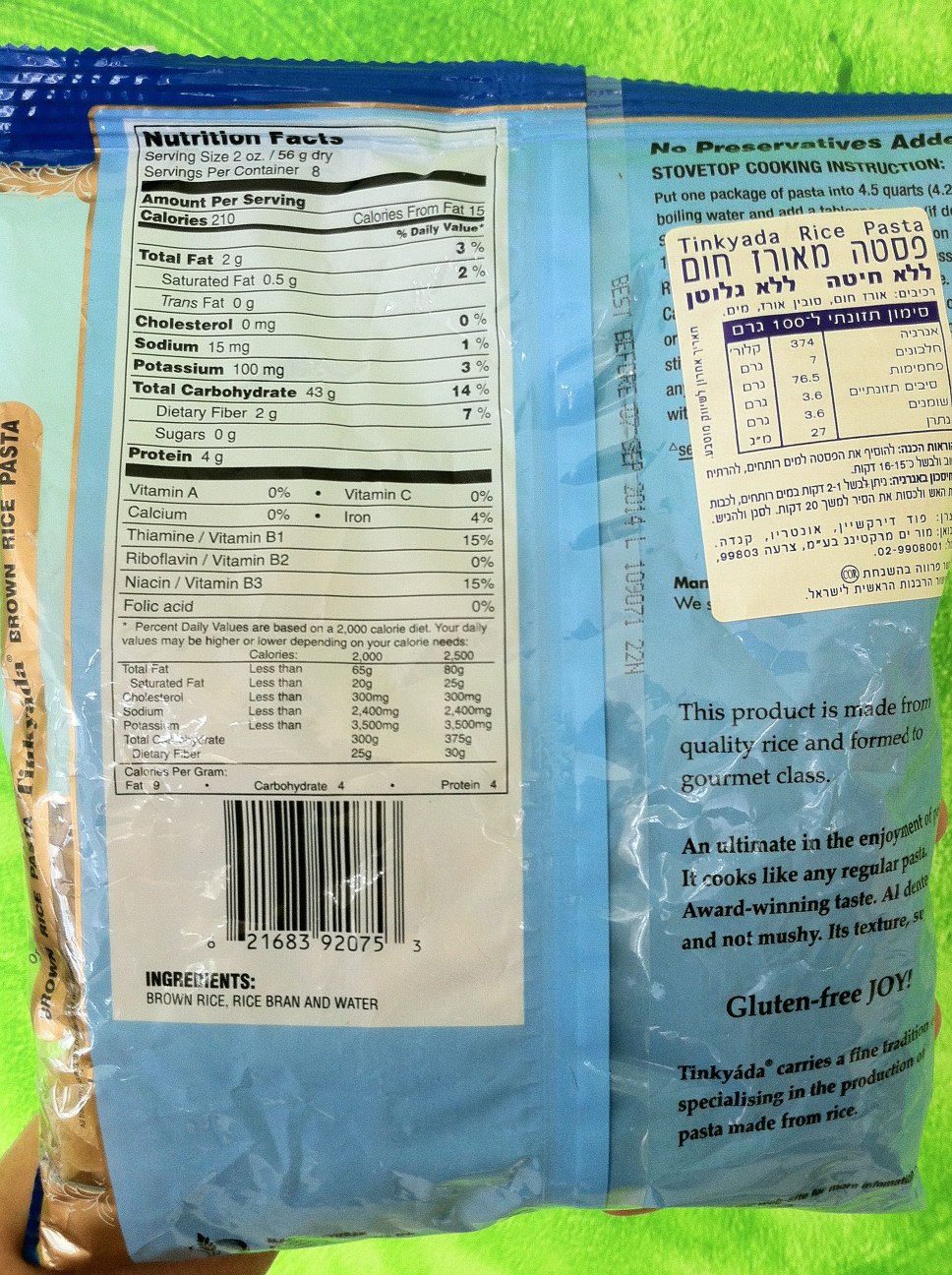This is a photograph taken indoors, showcasing the back of a blue package of Tinkyáda rice pasta. The left side of the package prominently displays the nutritional facts, detailing that each serving contains 210 calories, 2 grams of fat, 0.5 grams of saturated fat, 15 milligrams of sodium, 100 milligrams of potassium, 43 grams of carbohydrates, 2 grams of fiber, and 4 grams of protein. Adjacent to the nutritional information is some text on the right, accompanied by a white sticker that clearly states "Tinkyáda Rice Pasta." The rest of the text appears to be in another language. 

Towards the bottom of the package, it is noted that the product is made from quality rice and formed to a gourmet class, promising an ultimate enjoyment experience by cooking like regular pasta. The label also highlights that the product has an award-winning taste, is not mushy, has a good texture, and is gluten-free. The ingredients listed include brown rice, rice bran, and water.